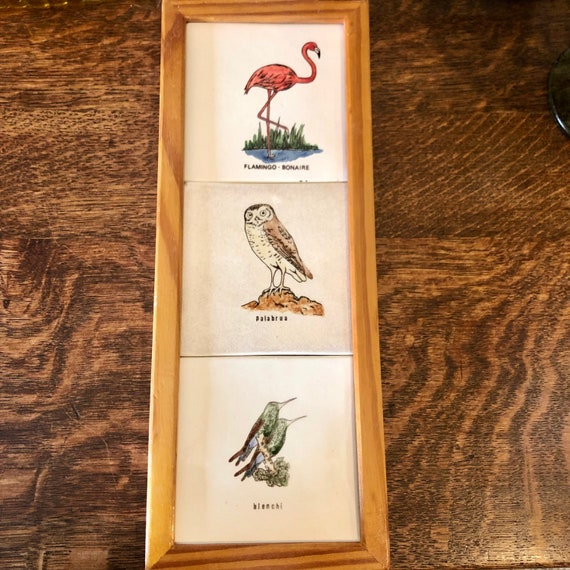This is a highly detailed photograph capturing a framed set of three artistic, colored sketches of birds, stacked and situated on a wood grain surface. The frame is made of a light or blonde wood. The top artwork features a pink flamingo, standing gracefully in some grass with one foot in the water, set against a white background. The text below this sketch reads "Flamingo Bonaire," although it is somewhat blurred in the image. The middle illustration portrays a brown and white owl standing on a yellow rock, also set against a white background. The text accompanying it is out of focus, but the bird strongly resembles an owl. The bottom sketch includes two hummingbirds with green, brown, and blue feathers, positioned on a stick. The text beneath this image is also unreadable. Each bird is vividly illustrated on individual tiles, which are framed together in this elegant arrangement.